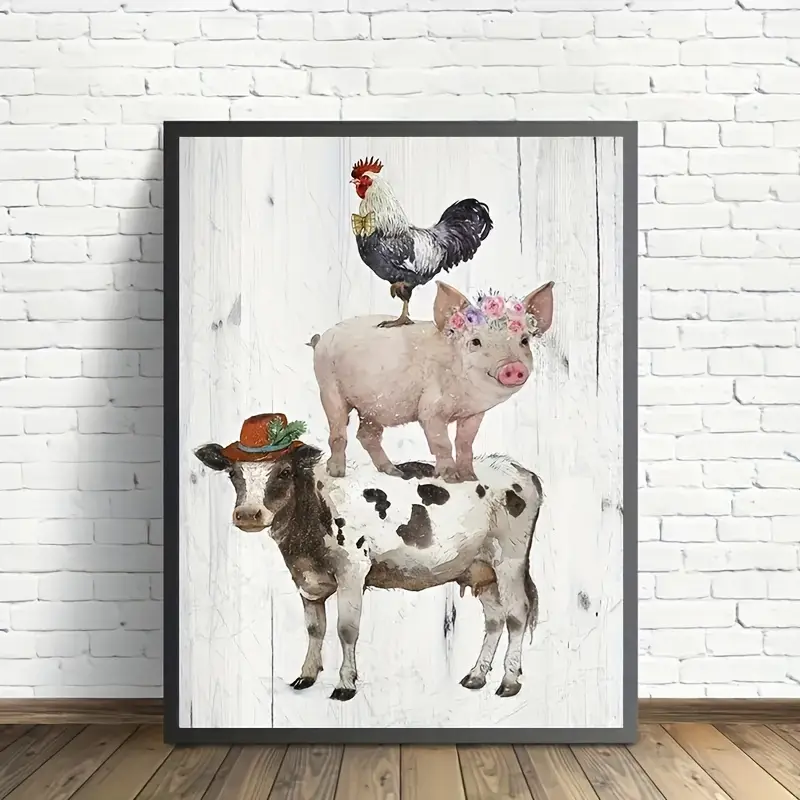The photograph captures a square-shaped painting propped against a white-painted brick wall with visible old brick texture beneath the paint. The scene is set on a dark, wood-plank floor with matching wooden baseboard trim. The painting features a black or dark gray frame and a background resembling vertically-planked barn wood, meticulously painted in light gray with knots and lines for a realistic texture. 

At the bottom of the depicted scene is a dairy cow, facing left, adorned with a German alpine hat featuring a headband, a little plume feather, a green feather, and a blue band. Standing on the cow's back is a cheerful pink pig facing right, wearing a garland or tiara of flowers in shades of pink, purple, blue, and white. At the top, a traditional black and white rooster faces left with a bright red comb and a black plume of a tail, one leg raised, and sporting a yellow bowtie. The combined elements of the room and the whimsical farm animal pyramid create a charming rustic atmosphere.